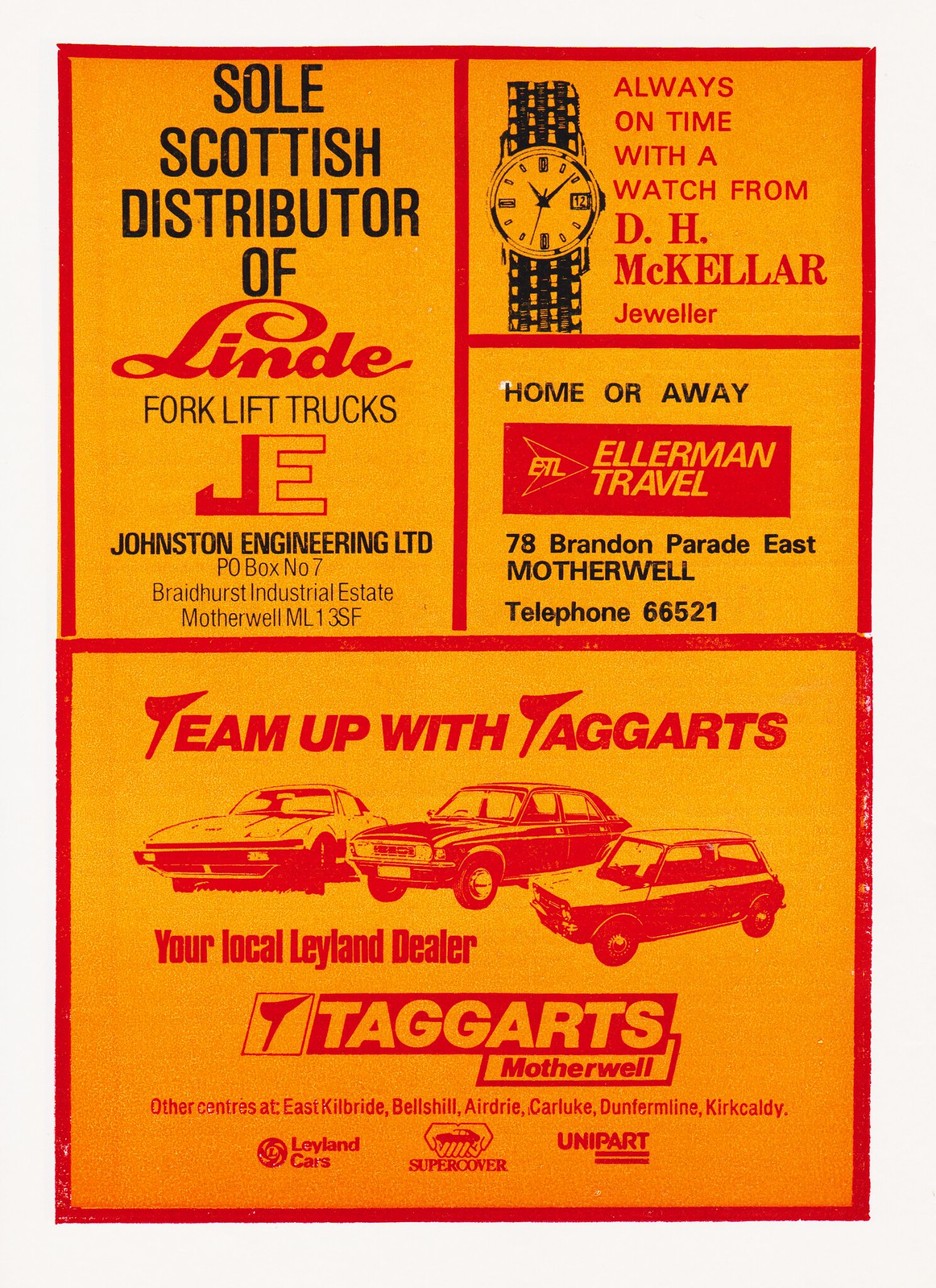The image showcases a detailed poster filled with a collage of various advertisements, featuring a deep yellow background and a red border encompassing the entire poster. Positioned in a structured manner, the poster has four main sections adorned with vibrant red text and distinctive logos.

In the top-left corner is an ad promoting the Scottish distributor of Lindell Forklift Trucks, detailing "J.E. Johnston Engineering Ltd, P.O. Bucks, N.O. 7, Branghurst Industrial Estate, Mother's Well, M.L. 13SF," accompanied by the Lindell and J.E. logos. Adjacent to this, in the top-right corner, there’s an ad with a watch image on the left and the slogan "Always on time with a watch from D.H. McKellar Jewelry" on the right.

Beneath that, another ad reads "Home or Away" with the Ellermann Travel logo, providing "7A Brandon Parade East, Mother Well, Telephone 66521." The bottom section of the poster features a larger advertisement promoting Taggart's, with the headline "Team Up with Taggart's." This ad showcases three pictures of cars and mentions "Your Local Leyland Dealer, Taggart's Mother Well," along with "Other Countries at East Kilbride, Best Shell, Airedale, Carluke, Dunstill, and Kirkcaldy." Three small, indecipherable logos are present underneath, adding to the poster's rich detail and vibrancy. 

The overall composition is well-organized, with a variety of colors including gray, red, orange, yellow, black, and white, evenly spaced across the poster, giving it an eye-catching and professional look, reminiscent of a page from a magazine.